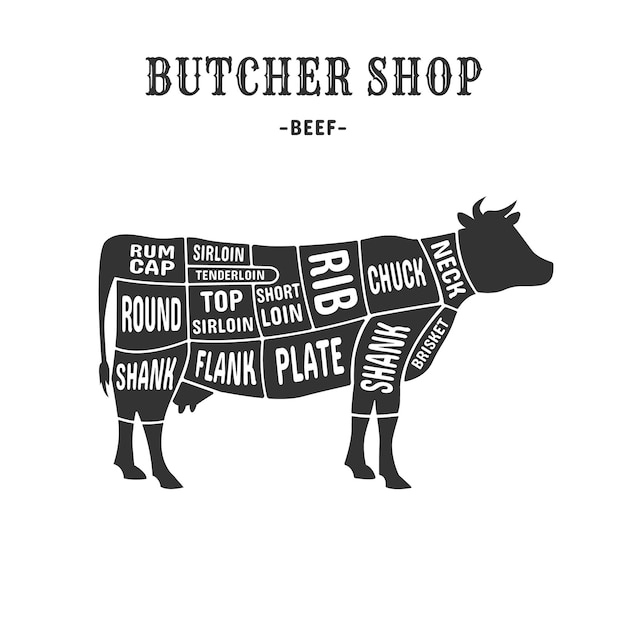The image is an illustration of a black silhouette of a cow, facing right, with white text detailing the various cuts of meat across its body, designed as a butcher's guide. At the top of the image, in an old-fashioned, calligraphy-style font, it reads "BUTCHER SHOP" followed by "BEEF" beneath it. The cow’s body is meticulously divided by white lines into labeled sections: starting from the rear, it includes the rump cap near the tail, the sirloin along the upper back, and the tenderloin beneath the sirloin. Moving towards the front, the short loin follows the sirloin, then the rib, chuck near the shoulder, and neck. Additional segments include the round beneath the rump cap, the top sirloin above the flank, and the plate lying forward of the flank towards the front legs. The terms “shank” appear on both the front and rear leg regions, and the brisket is indicated on the chest. The illustration is detailed and informative with clear, white text on a contrasting black silhouette, serving as a comprehensive butcher's diagram.